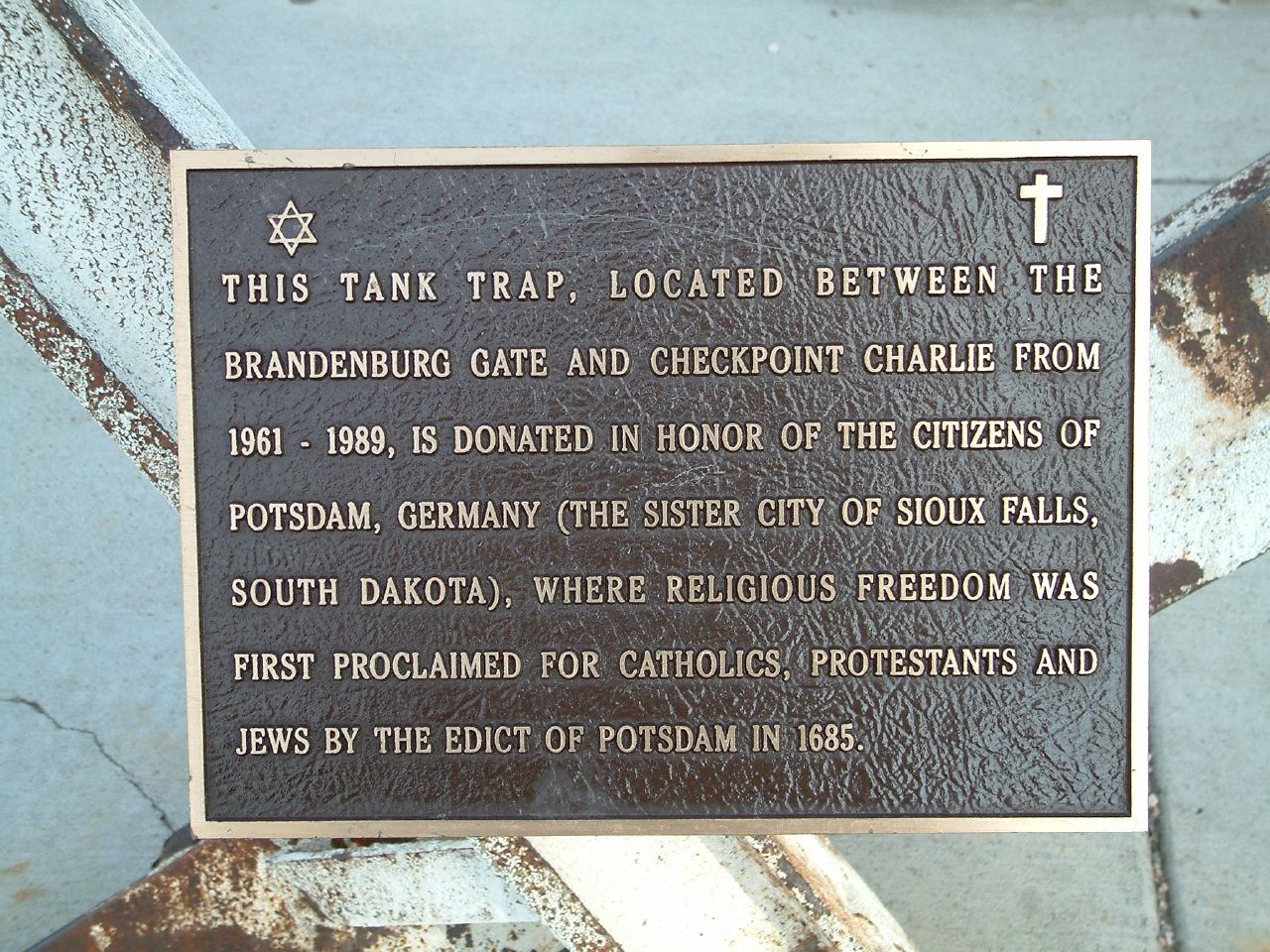The image depicts a detailed close-up of a metal plaque, potentially copper or some polished metal, bordered with a light brown or tan trim. The plaque, which is situated outdoors on what seems to be positioned against a wooden fence or wall marked with blue spray paint, features a Star of David in the upper left-hand corner and a cross in the upper right-hand corner. The inscription on the plaque reads: "This tank trap, located between the Brandenburg Gate and Checkpoint Charlie from 1961 to 1989, is donated in honor of the citizens of Potsdam, Germany (the sister city of Sioux Falls, South Dakota, where religious freedom was first proclaimed for Catholics, Protestants, and Jews by the Edict of Potsdam in 1685)." The background of the image shows an ambiguous post, pole, or rock structure, adding to the scene’s historical ambiance.